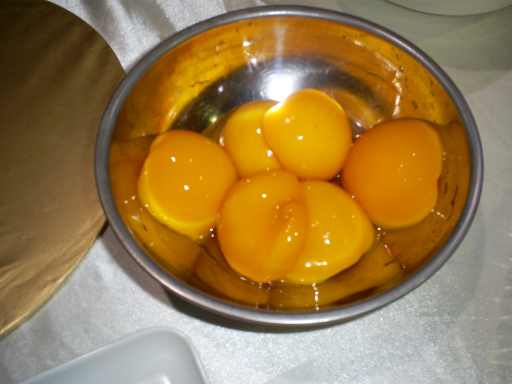This photograph captures a close-up view of a stainless steel mixing bowl on a white tabletop. Inside the bowl are six peach halves, likely removed from a can, glistening with syrup. These peaches appear to have been stewed, blanched, or boiled, giving them a tender and succulent texture. The light shining almost directly above is reflected in the steel bowl, casting a bright highlight on its surface. To the left of the bowl, a brown, wavy object, possibly a fabric-covered cutting board, adds a touch of contrasting texture. Additionally, the corner of a rectangular white plate or tray is visible peeking into the frame, enhancing the composition and providing context to the setting.